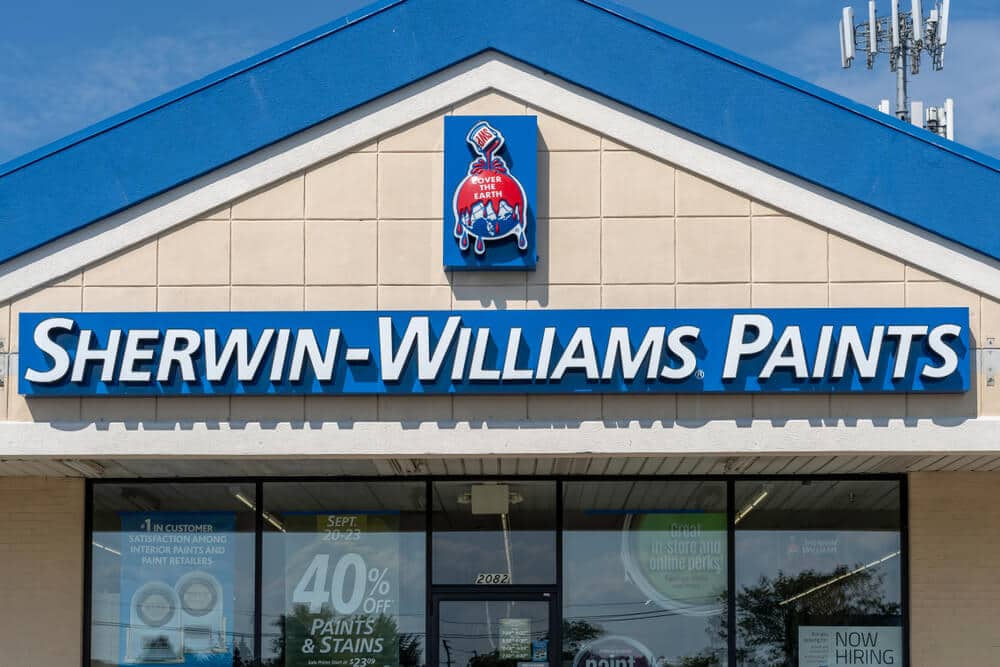This photograph captures the exterior of a Sherwin-Williams paint store. The facade features a striking 3D sign with "Sherwin-Williams" spelled out in large, white letters outlined in black, prominently mounted on a raised blue rectangle. Above this main sign is a smaller section of the building adorned with an arched, steepled rooftop that boasts white and blue trim, adding a touch of architectural interest.

Centrally placed above the main sign is Sherwin-Williams' iconic but controversial logo—an overflowing paint bucket with "SWP" on its side, spilling red paint to cover the Earth beneath it. The logo, rendered in 3D, protrudes from another blue panel, giving it added depth and visibility. The slogan "Cover the Earth," displayed alongside, adds to the logo's dramatic visual impact.

Below the signage, the building façade is dominated by glass. A central glass door is flanked by large floor-to-ceiling glass panels, all of which reflect the surrounding trees and power lines. Promotional signs in the glass windows advertise a significant sale on paints and stains, with discounts of up to 40% from September 20th to 23rd. This combination of architectural and promotional elements makes for a visually compelling and detailed storefront.